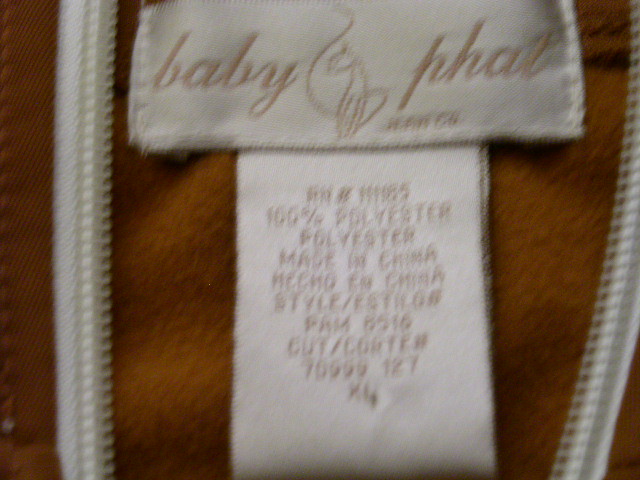This image, though blurry and of low resolution, depicts a square-shaped item with a zipper running along its edge. The zipper, which is white, is visibly positioned with sections on both the left and right sides. There are two distinct labels in the image: one at the top and another at the bottom. The upper label prominently displays the brand name "BABYPHAT" in pink-peach colored text set against a black background.